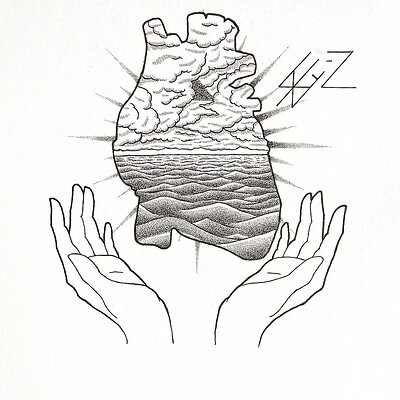This is a detailed pencil illustration of a feminine pair of hands, outlined and not fully detailed, stretched palms up at the bottom corners of the image. They create a receiving effect, almost like a basket. Above the hands, there is a black silhouette of a human heart, centered and prominent within the composition. The heart contains intricate details: the lower half resembles flowing sand dunes or waves in the sea that stretch to the horizon, while the upper half features an array of clouds. Light beams or starbursts radiate from the heart, enhancing its centrality. At the upper right of the heart, some inscriptions are present, notably including the letter "Z" and an X-like symbol with three horizontal lines cutting through it diagonally. The overall background of the image is off-white, adding a soft contrast to the black and white drawing.